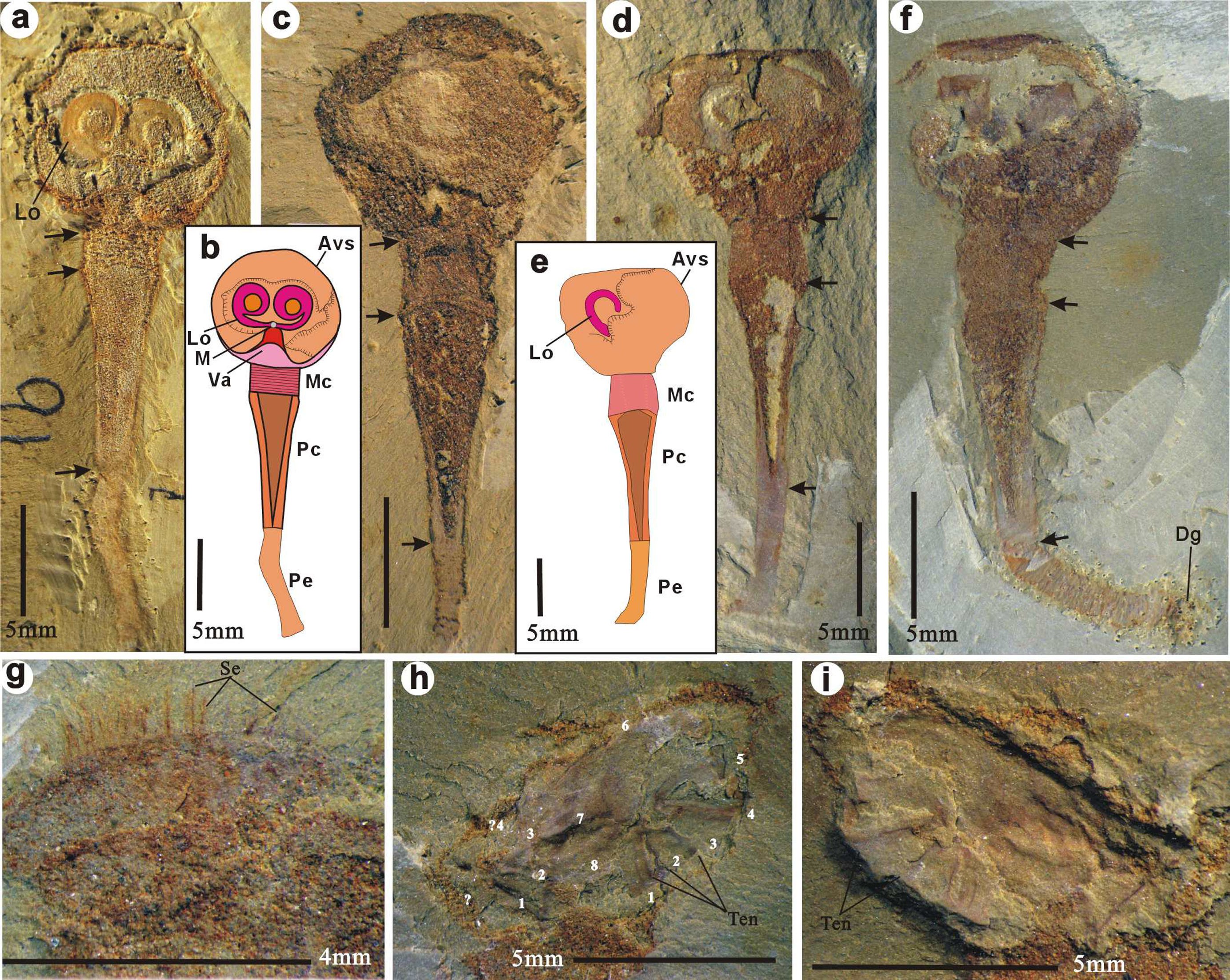The image is a horizontal, rectangular, educational diagram featuring fossilized remains. It is divided into two rows of photographs and sketches, each labeled with lowercase letters inside small white circles. The top row contains four images labeled 'a,' 'c,' 'd,' and 'f,' depicting a fossil with a circular top tapering to a point. The bottom row consists of three horizontal images labeled 'g,' 'h,' and 'i,' showing an oval-shaped fossil structure. Drawn cross-section images are set between the photographs, displaying the inner anatomy of the fossil and labeled with additional letters ('L,' 'O,' 'M,' 'V,' and 'A'). One of these sketches appears over the top images, specifically between 'a' and 'c,' and another between 'c' and 'd,' illustrating the presumed internal structure and dimensions of the fossil, which are indicated to be around five millimeters. The fossil somewhat resembles parts of a human body, including features that might be interpreted as a leg or a uterine structure.